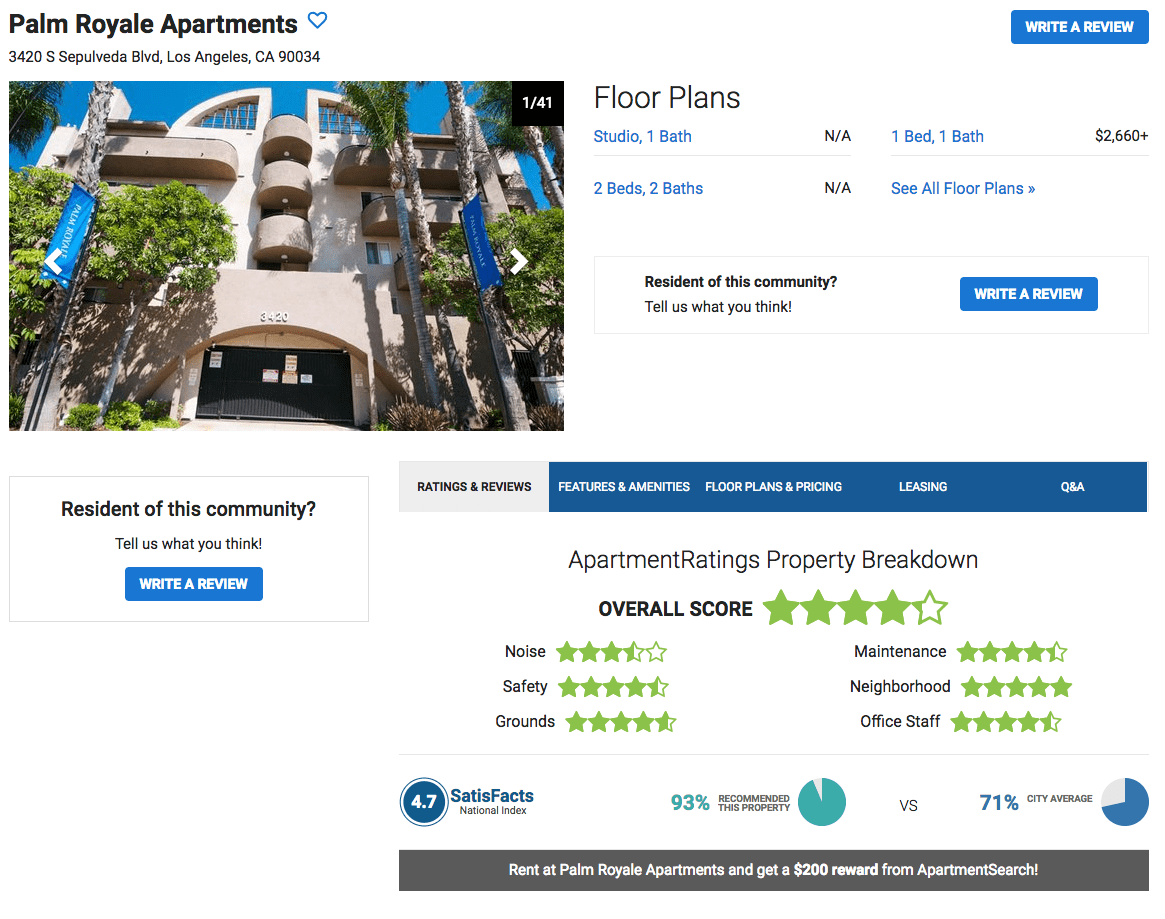This is a detailed screenshot of a listing from an accommodation booking site for Palm Royale Apartments, characterized by a clean, white background with blue accents for buttons. Prominently featured at the top left of the screenshot is the name "Palm Royale Apartments," accompanied by a blue heart icon. The address, "3420 South Superveda Boulevard, Los Angeles, California, 90034," appears just below the title. 

In the top right-hand corner, there is a conspicuous blue button labeled "Write a Review" in white text. Below the apartment's name, on the left side of the screen, a photograph showcases the front entrance of the building, with a striking view of palm trees and the building's facade.

Next to the photograph, a section titled "Floor Plans" lists various accommodation options: 
- Studio, one bath: Not applicable
- Two beds, two baths: Not applicable
- One bed, one bath: Starting at $2,660

A clickable link labeled "See All Floor Plans" is also available. Below this section, another prompt encourages residents to share their thoughts with the text, "Resident of this community, tell us what you think," followed by a blue button to "Write a Review."

On the right side, a navy navigation menu indicates that the current tab is "Ratings and Reviews" (highlighted in grey). Other tabs include "Features and Amenities," "Floor Plans and Pricing," and "Leasing and Q&A." Within the "Ratings and Reviews" section, the apartment complex is rated in various categories:
- Overall Score: 4 stars
- Noise: 3.5
- Safety: 4.5
- Grounds: 4.5
- Maintenance: 4
- Neighborhood: 5
- Office Staff: 4.5

Further down, three logos are displayed. A blue circle icon features a "4.7" rating from Satisfacts. Another icon shows "93%" in teal, indicating a high recommendation rate for the property compared to a "71%" city average depicted in blue. 

At the bottom of the screenshot, a dark grey block highlights a special offer in white text: "Rent at Palm Royale Apartments and get a $200 reward from apartment search!"